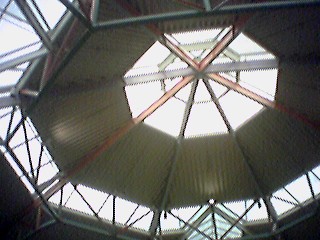The image captures an upward perspective of a glass and metal atrium ceiling inside a tall building, likely taken from the ground floor. The central focus of the photograph is a hexagonal pattern formed by large structural steel I-beams converging at the center, creating a star-like shape. The glass ceiling features a combination of gray, orange, black, white, and light blue hues, with natural light streaming through. The scene, set indoors during the day, resembles the expansive architecture typical of large atriums found in malls, complete with glass panels and additional structural supports around the edges. In the background, a triangular structure is visible, enhancing the geometric complexity of the design. The image is devoid of any text and highlights the spacious, open nature of the enclosure.